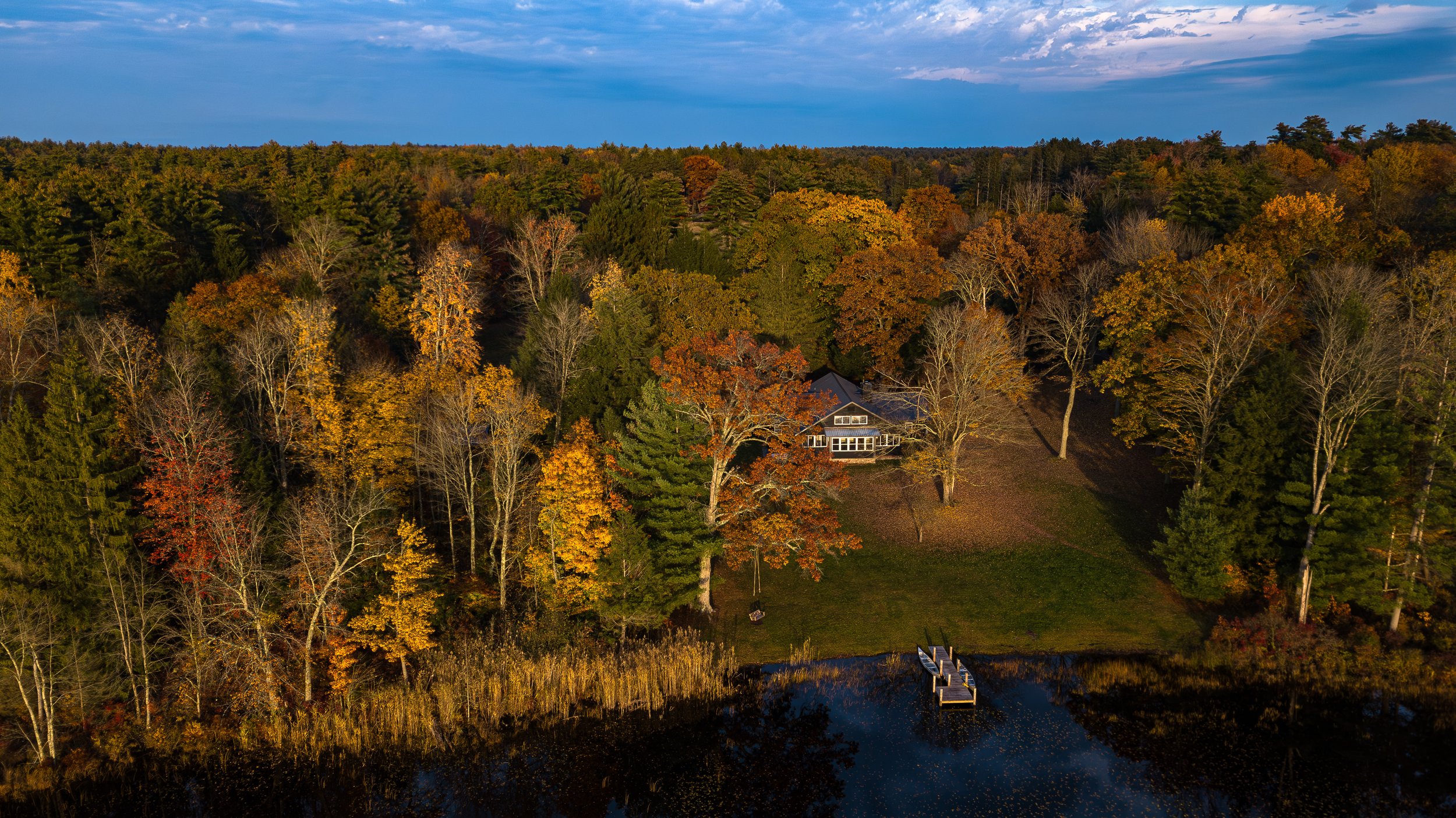The aerial image showcases a picturesque lakeside scene in the late fall, captured from treetop level, likely by a drone. Dominating the landscape are dense forests of deciduous trees with vibrant yellow, orange, and red foliage, intermixed with the evergreen hues of pine trees. A serene lake graces the bottom of the image, bordered by reeds and plant-based greens growing in the water. Extending from the shore is a wooden dock with a canoe and another small wooden boat.

At the center of the image is a small brown house with a triangular roof and an array of white windows, surrounded by a manicured lawn. A bare tree, stripped of its leaves, stands prominently in the front yard along with a few other scattered trees. The house is enveloped by the encroaching forest on both sides, creating a feeling of seclusion and tranquility.

The sky above is adorned with white clouds against a backdrop of either a blue expanse or dusk's dimming light, suggesting the photo was taken during the day with cloud cover or near sunset. The overall ambiance of the photo is calm and reflective, highlighting the natural beauty of the secluded lakeside retreat.